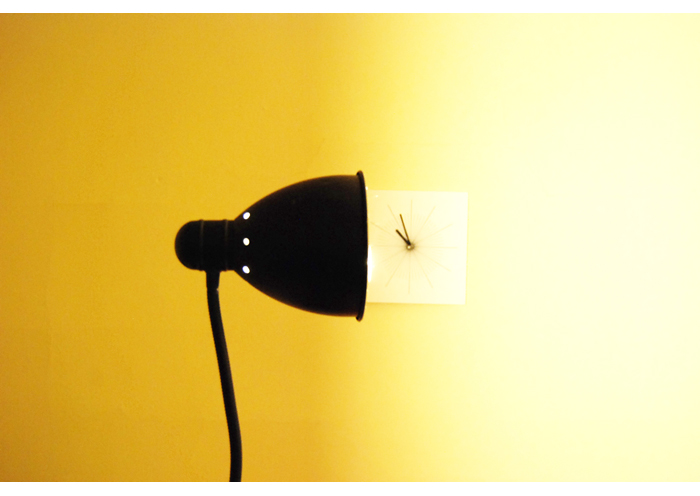The image captures a striking scene featuring a long, black gooseneck lamp with a cone-shaped head and drilled white vents, which is silhouetted against a two-toned yellow backdrop. The wall behind the lamp transitions from a dark, almost orangish-yellow on the left side to a lighter, almost white-yellow on the right. The lamp is turned on, casting bright illumination that highlights this gradient. Adjacent to the lamp, there is a square white clock with a sunburst pattern in the center. The clock displays the time as approximately three minutes to 11, marked by lines instead of numbers, with only an hour and minute hand. The lamp is positioned such that its light directly overlaps the clock, casting an intriguing shadow against the contrasting background.